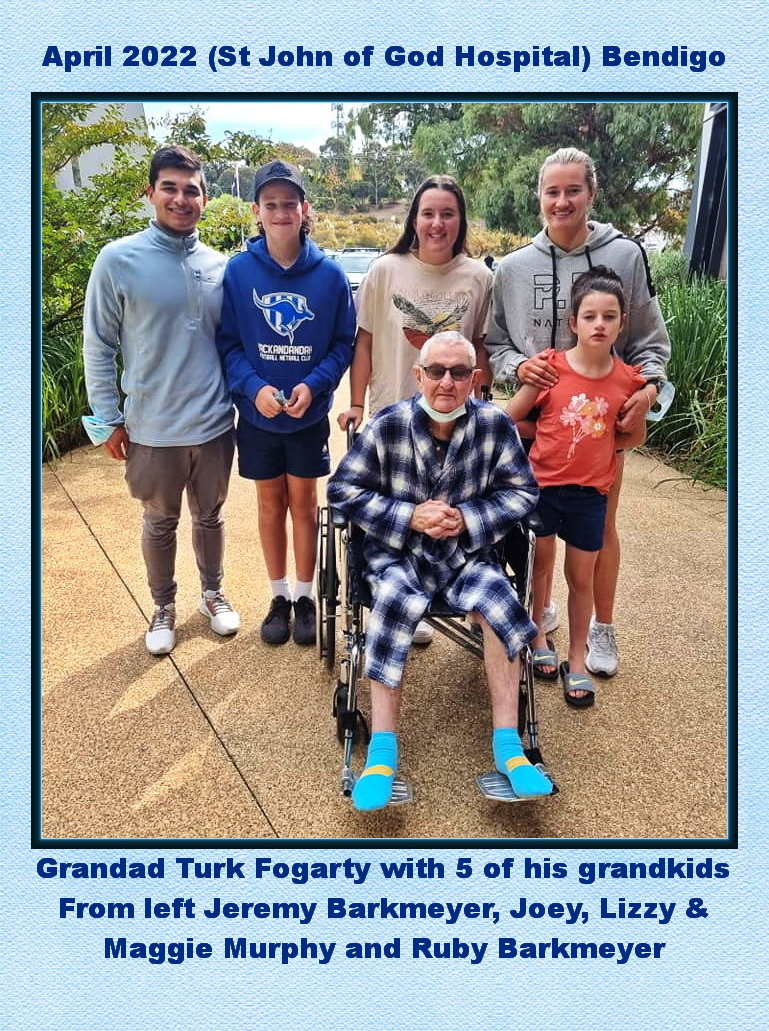This image features six people with a detailed caption in dark blue text above and below the picture, which is bordered by a light blue frame and a darker blue inner border. The elderly man at the center of the group is Grandad Turk Fagarty, seated in a wheelchair. He is dressed in a blue and white checkered robe and teal blue socks with yellow accents. He wears sunglasses and has a blue mask placed under his chin. His hands are clasped together, and he exudes a calm demeanor.

Grandad Turk Fagarty is surrounded by five of his grandchildren. Standing directly behind him from left to right are Jeremy Barkmeyer, Joey, Lizzie Murphy, and Maggie Murphy, with Ruby Barkmeyer standing in front of Maggie. The children appear to be in their 20s or younger. The setting seems to be outside a facility, possibly St. John of God Hospital in Bendigo, as suggested by the caption. The background includes various foliage against a paved, tan-colored ground.

The text above the picture reads: "April 2022 (St. John of God Hospital, Bendigo)," and the text below reads: "Grandad Turk Fagarty with five of his grandkids. From left: Jeremy Barkmeyer, Joey, Lizzie and Maggie Murphy, and Ruby Barkmeyer."